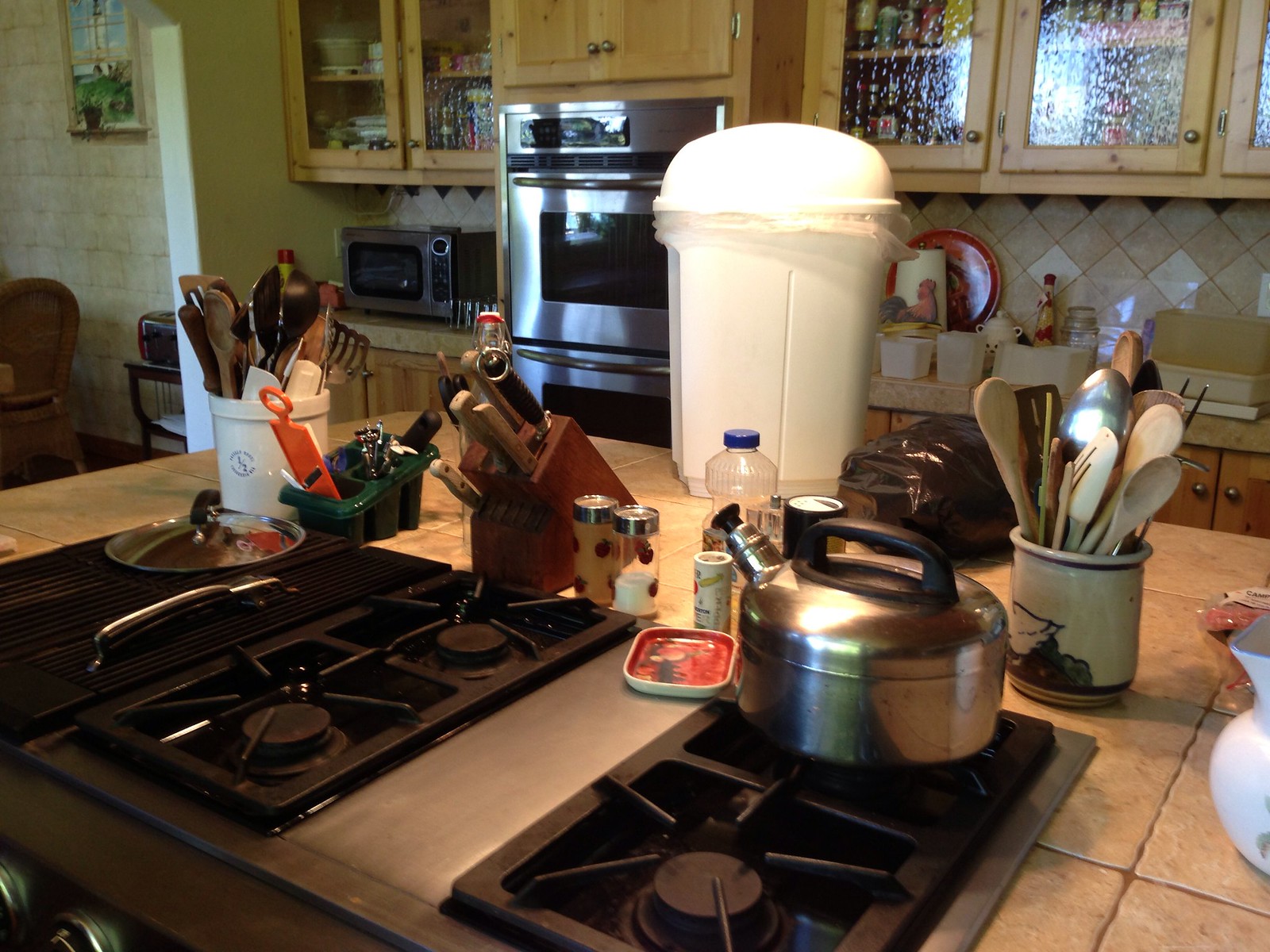In this photograph, the viewer peers slightly downwards at an angle onto a kitchen countertop, which extends diagonally upward to the left. The countertop consists of rough, beige-colored tiles, exhibiting a rustic charm. Centrally positioned on the counter is a square, silver stovetop featuring two black rectangular grates. Each grate is adorned with intricate, star-like spokes that converge at the center, marking the spot where the gas burners emerge. In the background, nestled between the stovetop burners, stands a large white plastic trash can with a domed lid, its contents secured by a trash bag that drapes over the edge. To the right of the stove, a Delftware canister, beautifully decorated in blue and white, brims with a variety of kitchen utensils, adding a touch of classic elegance to the functional workspace.